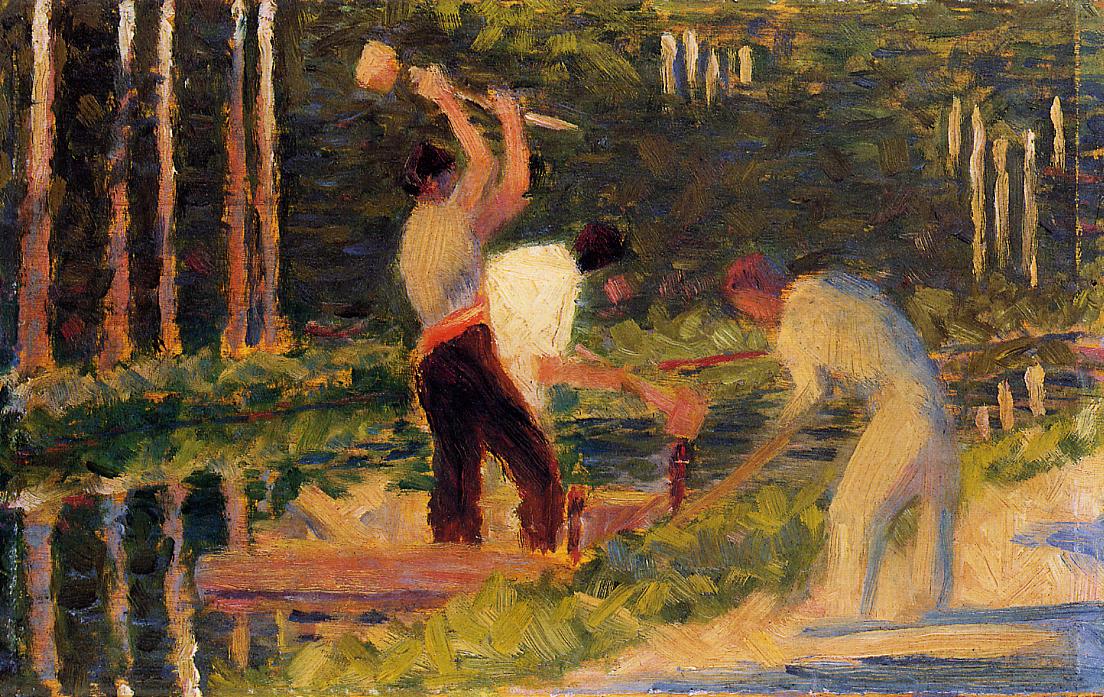This impressionist oil painting depicts three laborers working diligently on a dock or wooden structure by a narrow, reflective body of water, possibly a canal or riverside. The scene is set against a backdrop of dense, leafy trees, whose branches extend into the left corner and reflect in the water below, creating a serene natural ambiance. The central figure, clad in a white shirt and brown pants with a red belt, wields a large, rustic sledgehammer raised above his head, poised to strike. Partially behind him is another man, also in a white shirt, bent over and gripping a similar hammer, seemingly in the act of driving a post into place. On the opposite side stands a third worker, dressed entirely in white, assisting in the construction, possibly handling additional materials or tools. Vertical spikes and patches of grass further suggest the rugged, industrious setting of this vividly evocative painting.